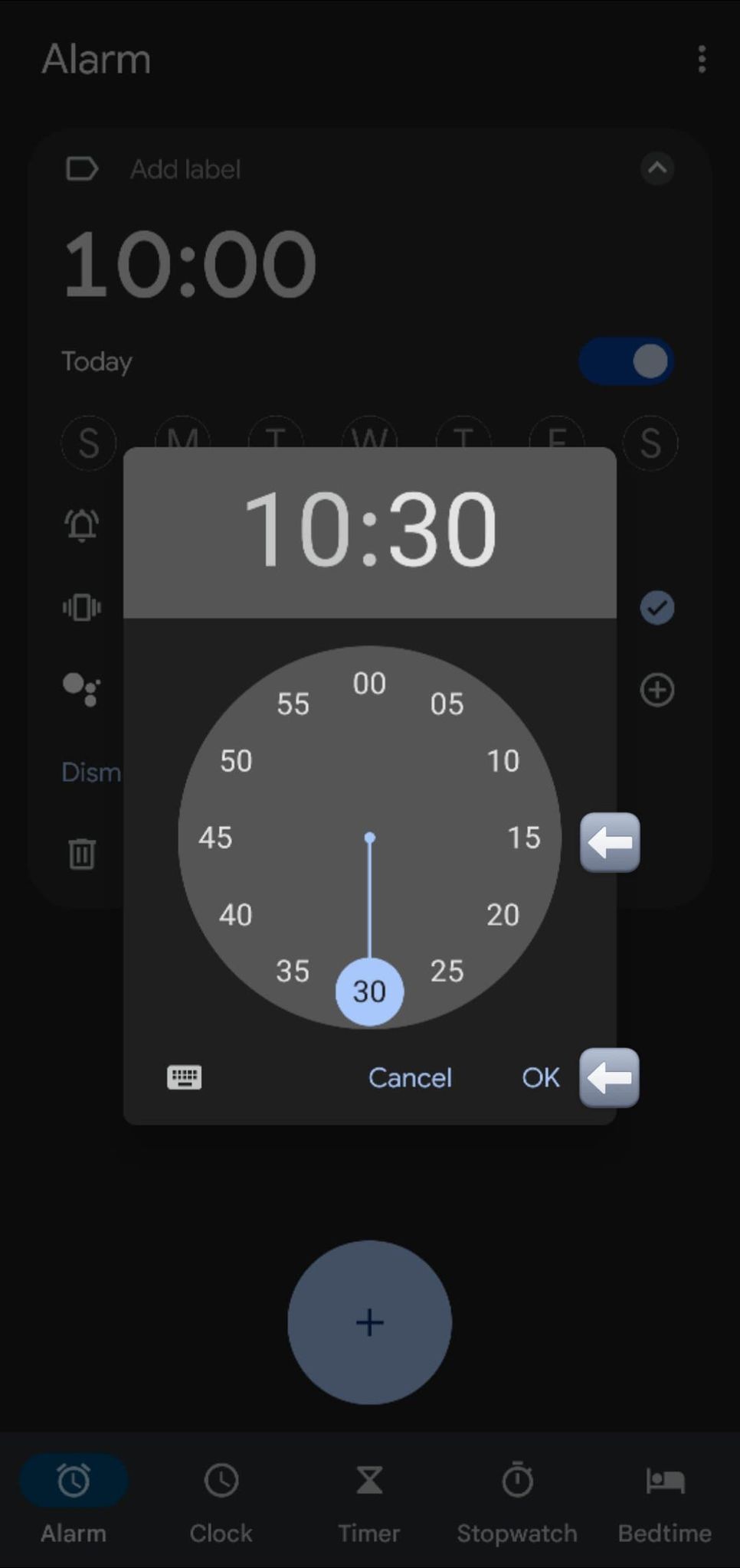This image is a screenshot from an alarm app on a mobile phone. Dominating the screen is a pop-up window displaying the settings for a countdown timer, specifically a stopwatch. At the top, the time is set to 10:30. Below that is a circular timer selection interface for setting durations from 0 to 60 minutes, with a blue circle highlighting the 30-minute mark. A slider bar allows for precise adjustments, and the blue circle is currently positioned at 30 minutes. The pop-up also features white arrows on a 3D light blue and gray square with curved corners, pointing at the timer and the OK button, though their purpose is unclear.

Below the timer, there are keyboard options and action buttons labeled "Cancel" and "OK." The rest of the screen displays a slightly shaded, blacked-out background, indicating the focus is on the pop-up.

In the background, the main app interface is partially visible. It shows the default "Alarm" tab active, with options to add labels and set specific times, days of the week (SMTWTFS), and alarm settings like vibration and dismiss. Icons for Google integration and a trash bin are also present. At the very bottom, there are navigation options: a plus symbol within a light blue circle, followed by tabs labeled Alarm, Clock, Timer, Stopwatch, and Bedtime. The Alarm tab is currently selected, explaining the prominent display of the pop-up in the center.